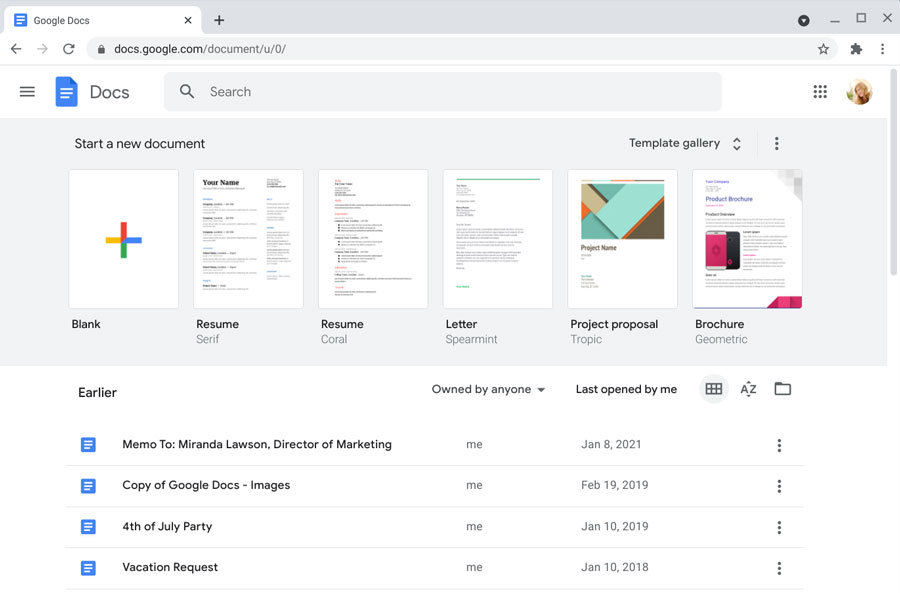The screenshot showcases the Google Docs home screen interface. At the top, a blue icon with white lines signifies Google Docs, accompanied by the text "Google Docs" in black. Below the icon, the URL "docs.google.com/document/u/0/" is displayed. Directly underneath, the word "Docs" appears alongside the same blue document icon, symbolizing Google Docs, and an avatar of a woman indicating a logged-in user.

The main part of the interface highlights the "Start a new document" section, featuring a template gallery. Users can initiate various documents including a blank one, two distinct resume styles, a letter, a project proposal, and a brochure. Each template is represented by a small preview image with an up and down arrow button located above for additional selections.

Further down, the screen displays a list of recent files accessed in Google Docs. The files shown include four documents with dates ranging from January 10, 2018, to January 8, 2021. The documents seem work-related, with titles indicating matters like a director-related document, a Fourth of July party plan, a vacation request, and an image file.